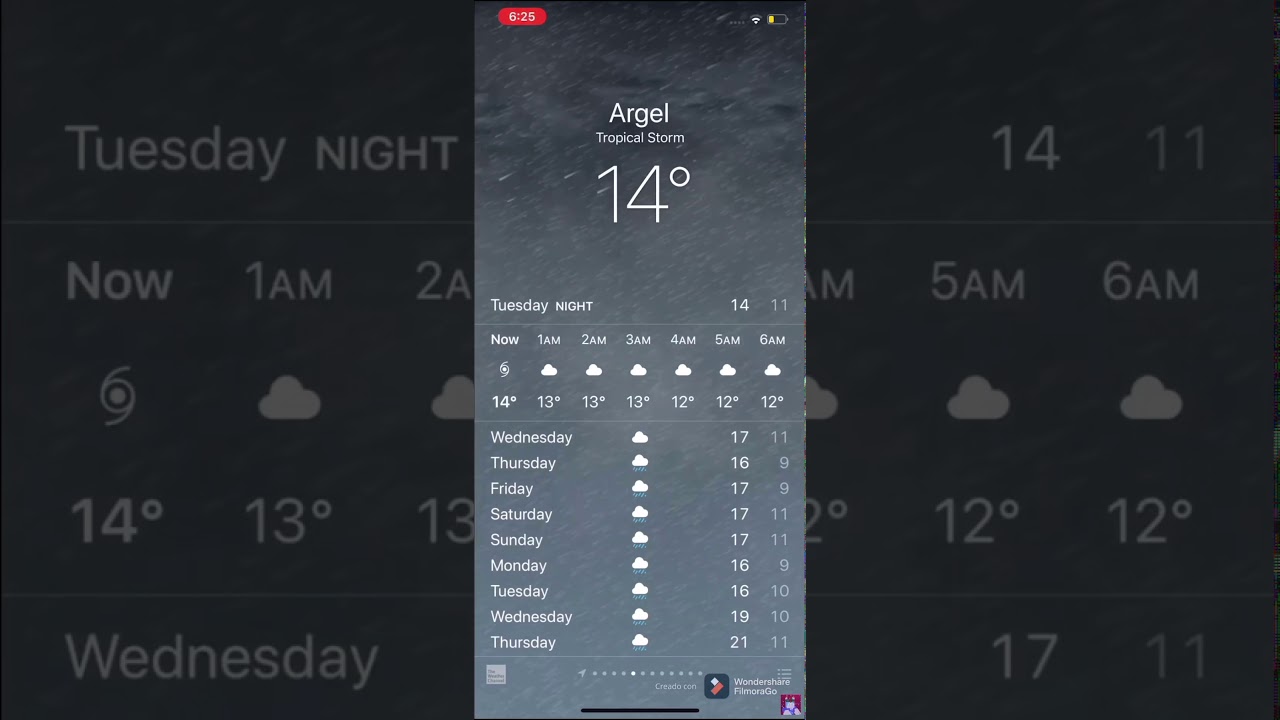This image is a screenshot of a weather app displaying the forecast for Argyle, highlighting a tropical storm condition. At the top of the screen, the current time reads 6:25 AM, with standard status icons for battery (which is slightly over halfway depleted and needs charging), Wi-Fi, and signal strength. 

In the main section, the current temperature is shown as 14°C amidst tropical storm conditions. Hourly forecasts are detailed below for Tuesday night transitioning into early Wednesday morning, showing consistent mostly cloudy conditions with temperatures as follows: 1 AM at 13°C, 2 AM at 13°C, 3 AM at 13°C, 4 AM at 12°C, 5 AM at 12°C, and 6 AM at 12°C. 

The daily forecast for the upcoming days is presented below, indicating continuous rain with the following temperature highs and lows:
- Wednesday: High of 17°C, Low of 11°C
- Thursday: High of 16°C, Low of 9°C
- Friday: High of 17°C, Low of 9°C
- Saturday: High of 17°C, Low of 9°C
- Sunday: High of 17°C, Low of 11°C
- Monday: High of 16°C, Low of 9°C
- Tuesday: High of 17°C, Low of 10°C
- Next Wednesday: High of 19°C, Low of 10°C
- Next Thursday: High of 21°C, Low of 11°C

At the bottom right corner, a watermark indicates the screenshot was created with Wondershare FilmoraGo. The app is meticulously designed to provide detailed weather information, including current conditions, hourly updates, and extended daily forecasts.